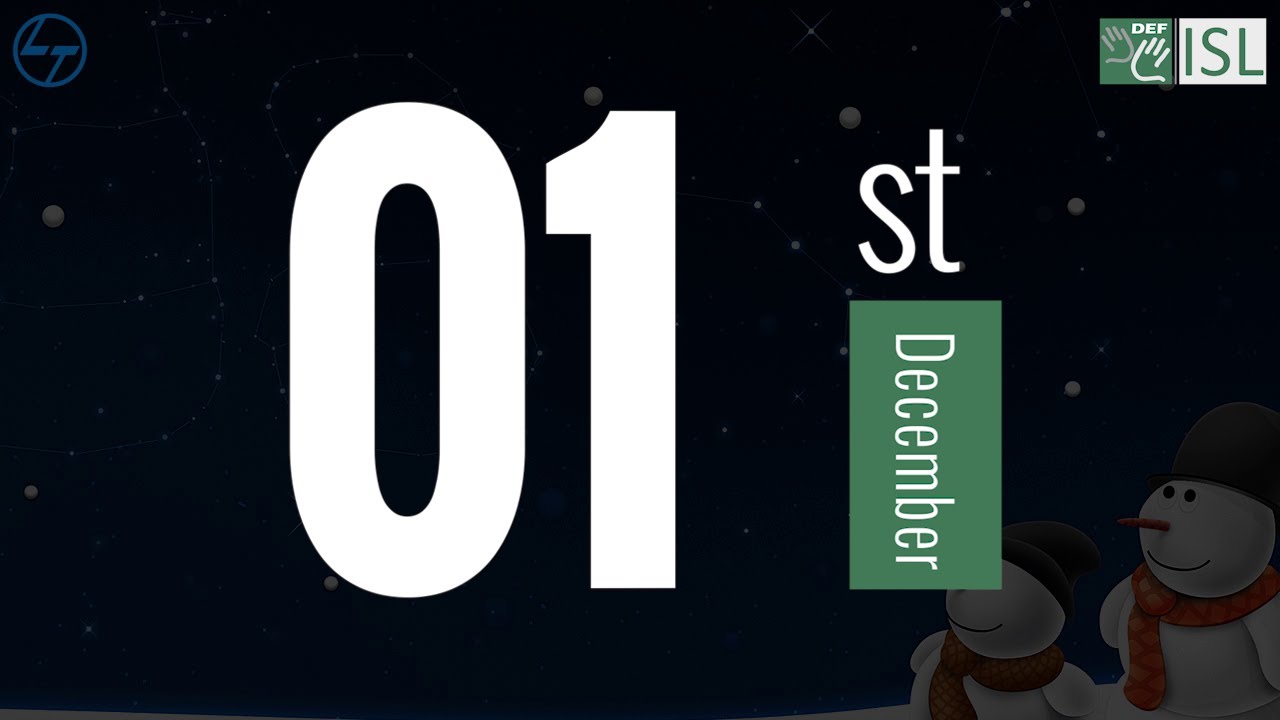The image appears to be a festive, winter-themed calendar announcement for December 1st. The background is predominantly a dark, almost black sky speckled with white dots that resemble falling snow. In the bottom right corner, two cheerful snowmen gaze upwards towards the sky. The snowman to the right is slightly taller, and both are adorned with cozy scarves and traditional carrot noses, bringing a sense of warmth and joy to the scene.

In the center of the image, a large "01" is prominently displayed, followed by "ST DECEMBER" with the "DECEMBER" vertically aligned within a green rectangle. This effectively emphasizes the date and month. In the upper left corner, a blue circle featuring the letters "LT" is visible. In the upper right corner, there is a green square with two hands inside it, labeled "DEF." Additionally, a white square displaying the letters "ISL" can be seen.

Overall, the image uses a combination of elements to convey a festive spirit, marking the first of December with holiday charm.